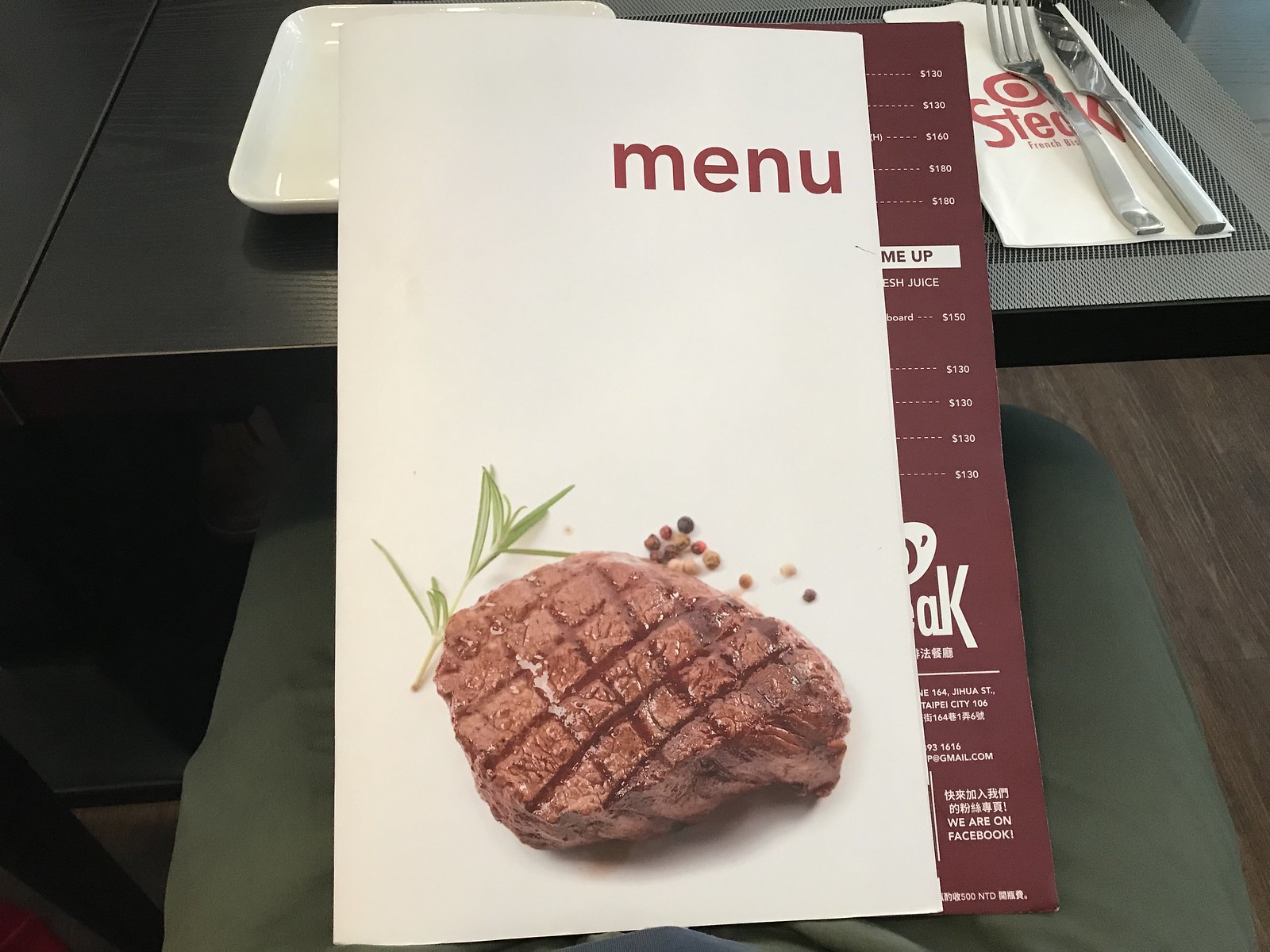In the photograph, a rectangular menu with a white plastic backdrop is being held in someone's lap as they sit at a dining table. The individual, who wears green pants and appears to have a slender build, has legs visible in the shot, but their gender is indeterminable. A white shoe can be seen under the table, likely belonging to a dining companion seated across from them. 

The menu's front cover showcases the word "Menu" in maroon font, succinctly placed above a tantalizing image of a grilled steak, complete with distinctive grill marks. The steak appears juicy and is garnished with whole peppercorns and a sprig of an herb, perhaps rosemary.

Due to the shorter front cover, part of the interior pages of the menu is visible, revealing prices such as $130, $160, and $180, along with a small logo design. Chinese characters are also discernible, suggesting the menu features Asian cuisine. The menu leans against a table with a black tabletop, and on the table, a white square plate accompanied by silverware is neatly arranged.